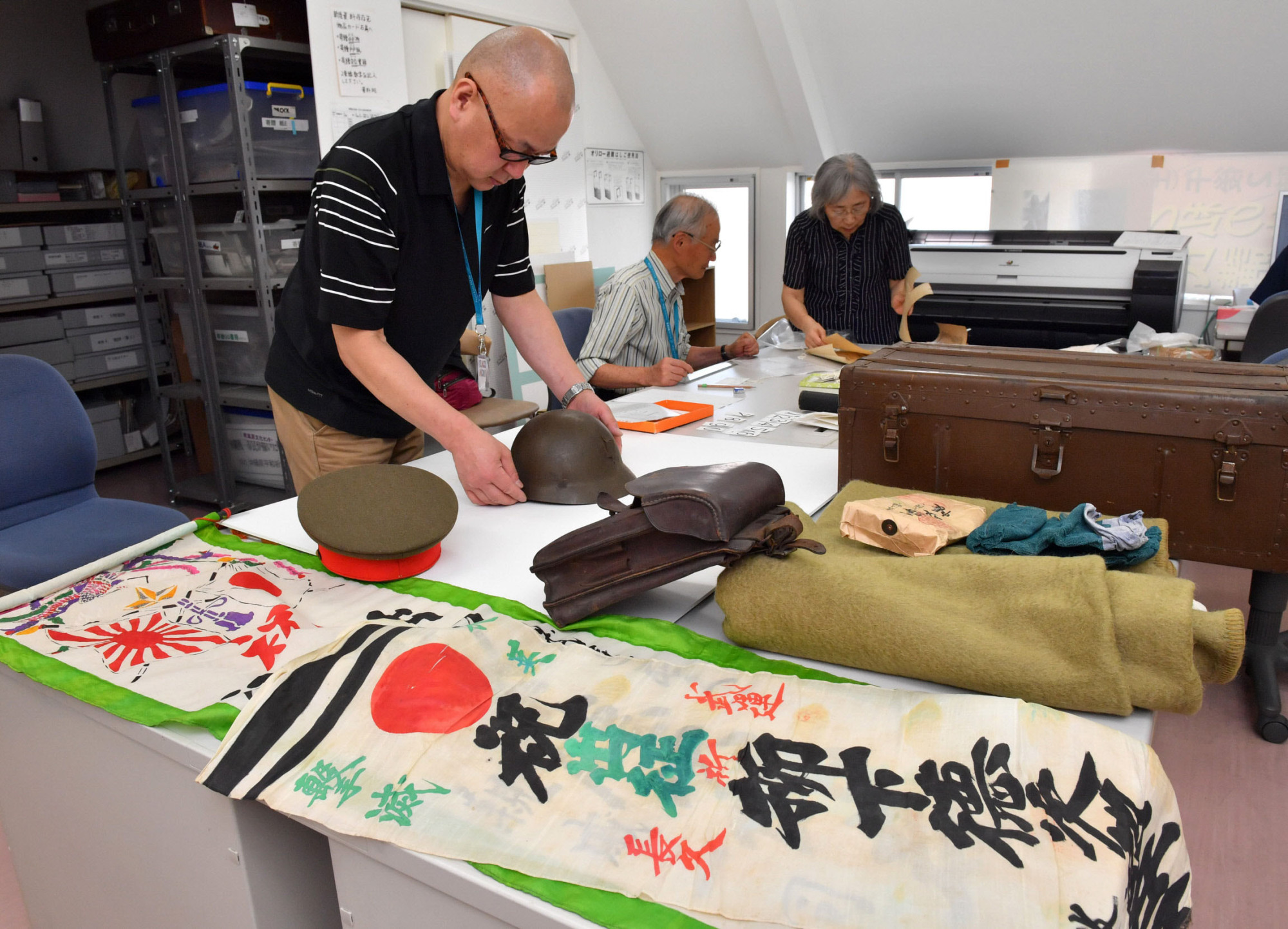In this image, three Japanese historians are gathered in a white room engrossed in examining World War II artifacts. A bald man with black glasses, wearing a navy blue shirt with white-striped sleeves and khaki pants, stands over a large working table. He is closely inspecting a mix-metallic military hat from the era. Around the table, which is covered with various memorabilia, is an older man and woman, both with gray hair, sitting and poring over pages alongside an array of items. A white banner with oriental print featuring a red circle resembling the Japanese flag is prominently displayed on the table. A leather backpack sits near a cloth military cap. The table also holds an olive green blanket with additional pieces of fabric and what appears to be an old, possibly war-time, trunk. Gray metal shelves stacked with various bins and items line the background of the room, suggesting an environment rich in historical research materials.